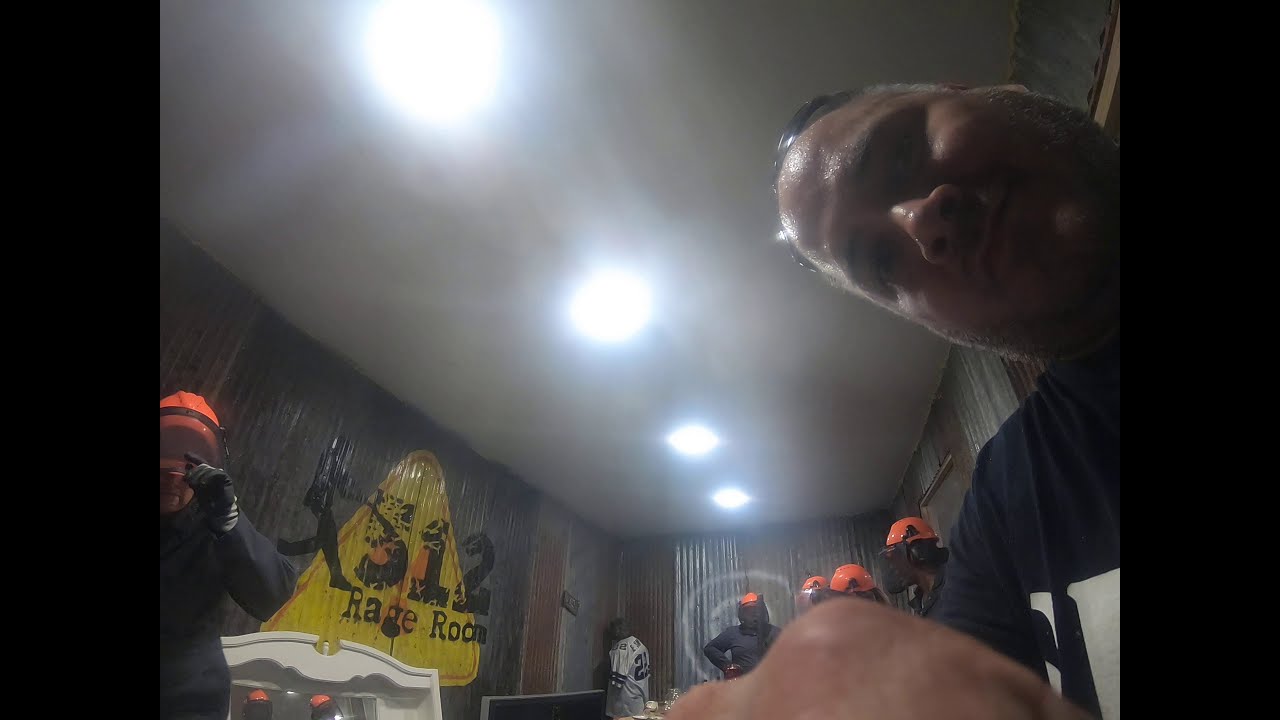The image depicts a scene inside a large, commercial Rage Room, identified by a prominent black drawing of a man and the text "512 Rage Room" against a yellow triangle on the back wall. In the foreground on the right, there's a middle-aged white male in a dark blue shirt, looking down seriously at his phone. Directly behind him are several people equipped with orange helmets and blue jackets, typical protective gear for this kind of activity. One individual in an orange helmet and black jacket stands near the left wall, alongside a mannequin dressed in what appears to be a football jersey numbered "2." The room is brightly illuminated by ceiling lights, and features industrial elements like corrugated metal surfaces. Just below the "512 Rage Room" text, a white cabinet is partially visible, suggesting objects that participants might smash during their session. The setting gives a sense of a controlled environment where individuals, like those pictured, can engage in stress-relief activities by smashing various items.